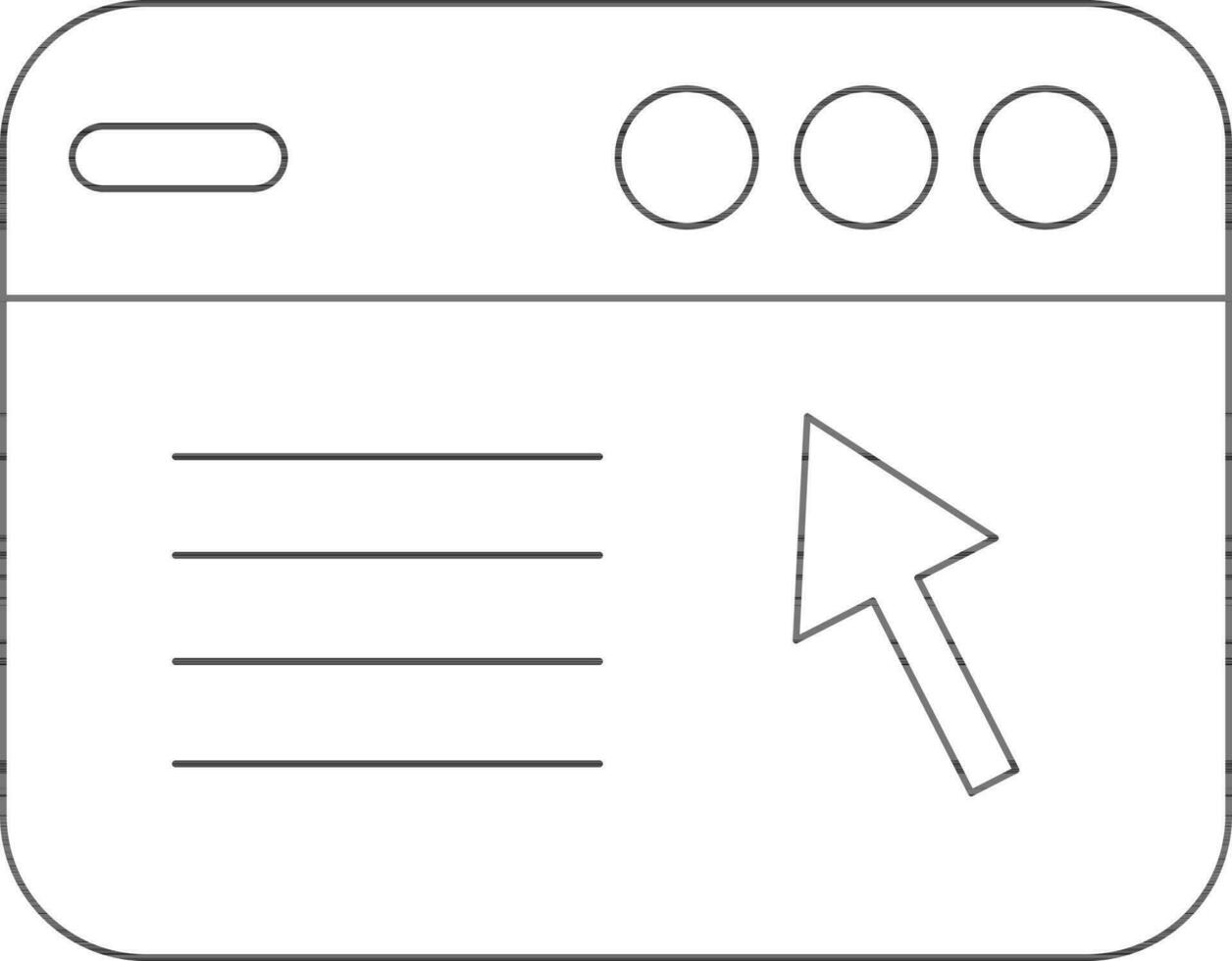The image depicts a simple rectangular nametag graphic featuring various elements. The outer rectangle has slightly curved corners, and its top and bottom sides are twice as long as its left and right sides. The interior is divided into two sections by a horizontal line. In the upper section, there are three white circles with black borders located in the upper right corner, and an oval-shaped, pill-like figure with rounded edges on the upper left side. In the lower section, four short horizontal lines are positioned on the left side, presumably for text input. To the right of these lines, there is an arrow symbol pointing diagonally towards the upper left. The background within this inner rectangular area is predominantly white.